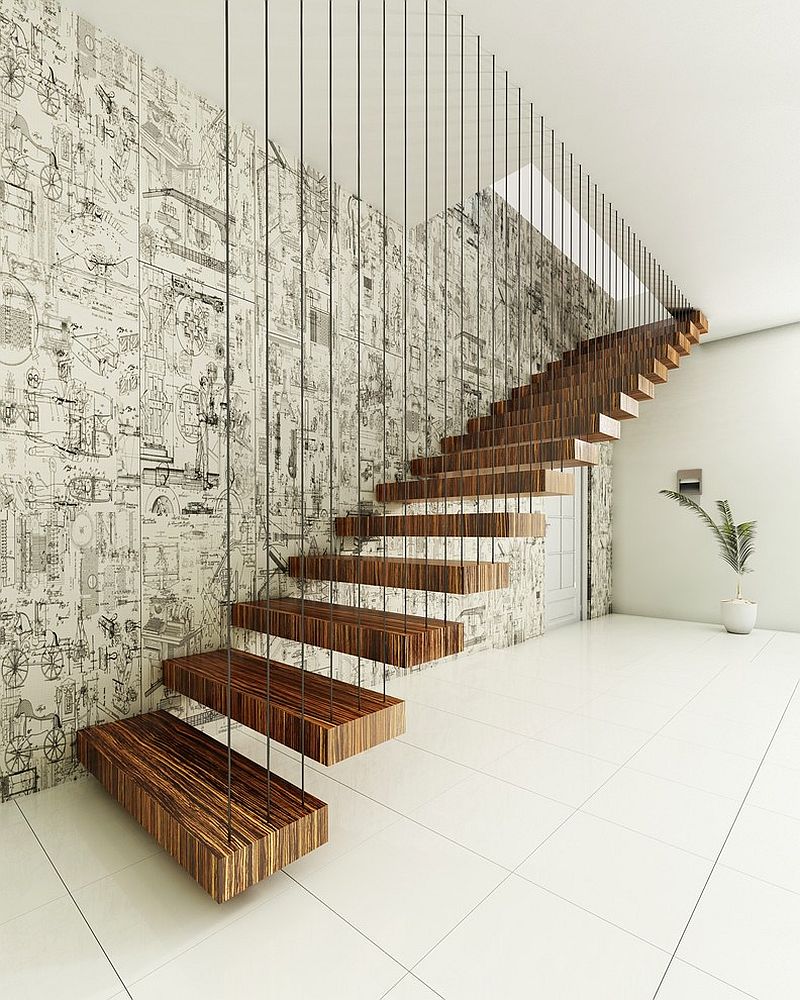The image depicts a striking open or floating staircase, seemingly inside a large foyer, potentially within a house or office complex. The staircase is suspended from the ceiling by sturdy steel wires, giving the impression that the wide, thick wooden steps are floating. These steps exhibit a textured grain with varying wood colors. The flooring beneath is white tile, extending into an entrance where a large plant in a white pot stands prominently. The staircase ascends beside a wall adorned with busy black-and-white wallpaper featuring an eclectic mix of diagrams, including bicycles and horse designs. Beneath the staircase, there is a door that adds to the functional yet stylish layout of the space. The lack of a banister further emphasizes the modern, minimalist design of this architectural feature.